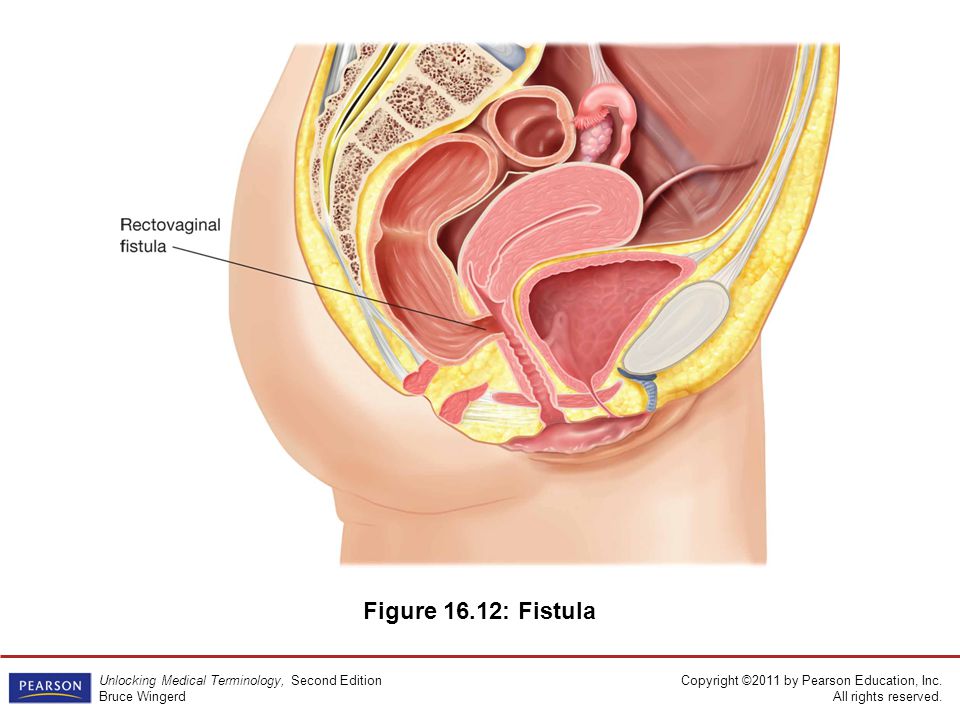The image is a detailed medical diagram, specifically a cross-sectional side profile of the female pelvic region, illustrating a rectovaginal fistula. Central to the illustration, various anatomical structures such as the uterus, fallopian tubes, ovaries, bladder, and rectum are clearly depicted. The diagram employs a range of colors including pink, yellow, teal, peach, orange, white, and black to differentiate the organs and tissues. Black arrows and labels are strategically placed to identify the rectovaginal fistula, an abnormal connection between the rectum and vagina, with simple black lettering for clarity.

Accompanying the diagram, the text includes "Figure 16.12 - Fistula," and credits Pearson's "Unlocking Medical Terminology, Second Edition" by Bruce Wingerd, with a visible copyright noting "2011 by Pearson Education, Inc., all rights reserved." The image's setting suggests a medical or educational context, providing a comprehensive visual aid for understanding this medical condition.